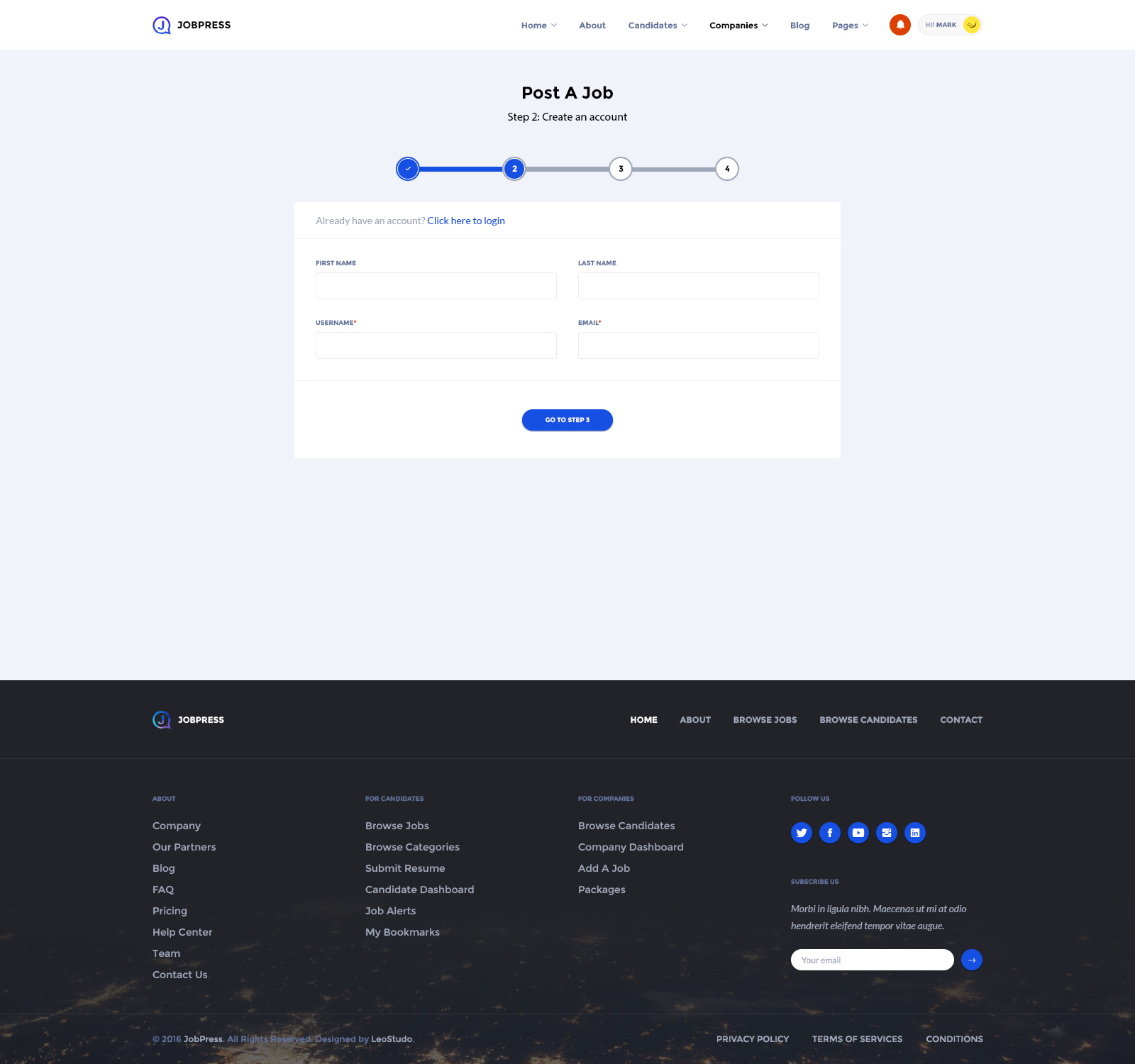The image appears to be a detailed screenshot from a job posting website. At the top of the page, there is a thin white line. On the left side of this line is a blue circle containing a white 'J'. Next to the circle, the text "Jaw Press" is written in black. To the right, a navigation menu displays items in black text: "Home" with a drop-down arrow, "About," "Candidates" with a drop-down arrow, "Companies" (which appears bold) with a drop-down arrow, "Blog," "Pages" with a drop-down arrow. Additionally, there's a red circle featuring a white bell icon. 

Below this navigation menu, there exists a subtle, pale light blue background. At the center top of this section, the bold text reads "Post a Job." Below this, the step "Step 2: Create an Account" is indicated. Further down, there are four connected circular icons indicating steps: 
1. A white circle containing the number '1', 
2. A blue circle containing the number '2' in white, 
3. A gray bar leading to a white circle with the black number '3', 
4. The gray bar continues to another white circle with the black number '4'. 

Beneath this sequence, there's a white text box bearing the gray text "Have an account?" followed by a blue clickable link "Click here to log in."

The user input section follows, starting with "First Name" in black next to an entry bar, and then "Last Name" similarly with an adjacent input field. Below these, "Username" and "Email" each have a line for input.

At the bottom of this section, there is a blue bar with white text saying "Go to Step 3." Near the footer, a black bar contains white text listing "Job Press," "Home," "About," "Browse Jobs," "Browse Canada," and "Contact."